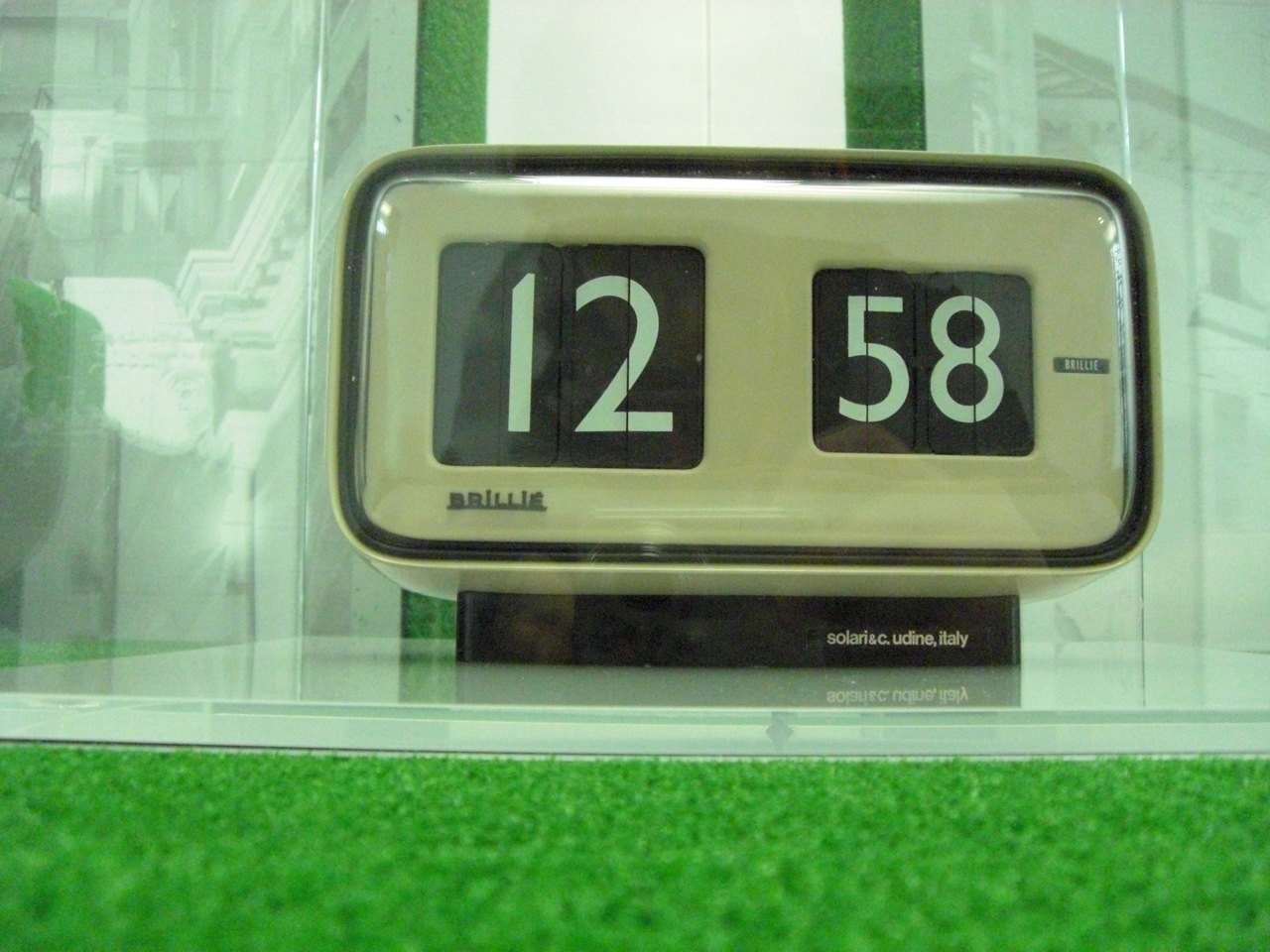This photograph features a vintage-style clock encased behind a protective glass or plastic enclosure, possibly situated within a shopping mall or an atrium given the visible architectural elements such as buildings, steps, and windows in the background. The clock, which bears the brand name "BRILLE," prominently displays the time as 12:58. The design of the clock is quite unique, with a rectangular beige face framed by black trim and accompanied by a black base. Instead of a digital display, this clock showcases an old-fashioned flip mechanism where white numbers on black backgrounds are used to indicate the time. The base of the clock also has some white writing on the right side, adding to its vintage charm. The foreground of the image includes a strip of green astroturf or grass covering roughly a fifth of the photo's height, flanked by two vertical green turf bars that rise up behind the clock, offering a striking contrast to the mechanical and architectural elements within the enclosure.